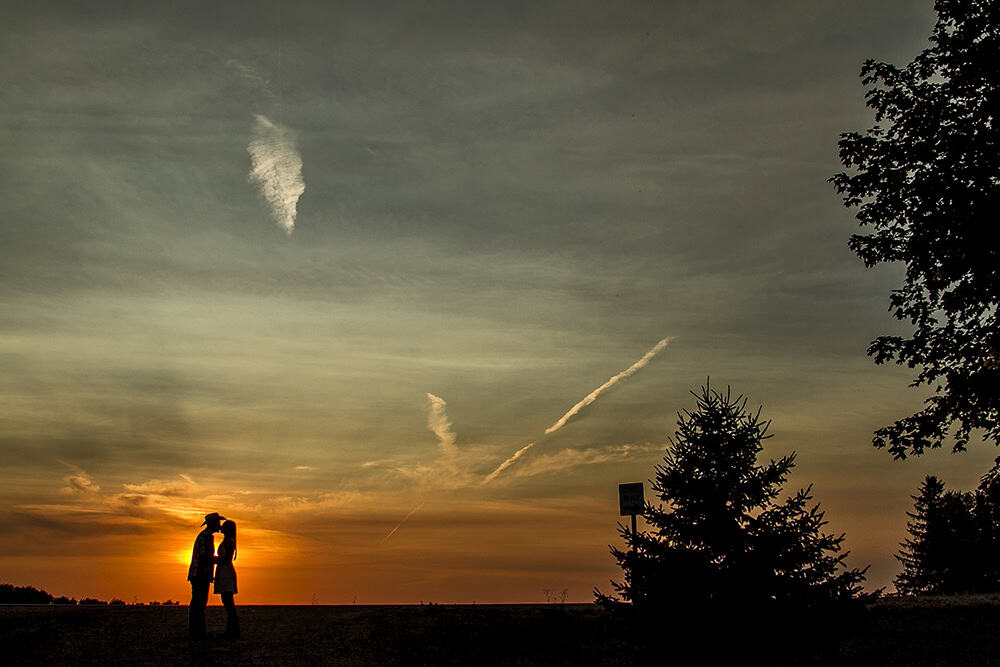In this evocative sunset photograph, the sky is a hazy blend of bluish-gray with streaky gray clouds, dramatically lightening to an orange and gray band near the horizon where the sun emits an orange glow. Against this vivid backdrop, the black silhouette of a couple kissing stands prominently. The man wears a cowboy hat and jeans, while the woman, with long hair, dons a dress that falls just above her knees. Their intimate moment is framed by scattered streaks of white clouds and noticeable jet streams above. To the right, silhouettes of trees and a street sign suggest a countryside setting, adding depth and context to the tranquil scene.